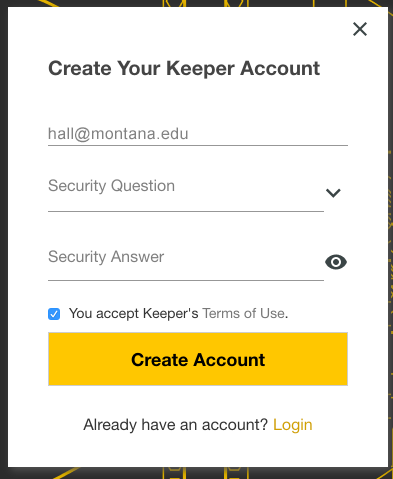The image depicts an account creation page for Keeper, featuring a clean user interface within a central white box set against an intricate gold and black patterned background.

At the very top right corner of the white box, there is an ‘X’ icon for closing the window. Below the title "Create Your Keeper Account," there is a field labeled "Email," pre-filled with an example email address (hall@montana.edu). This is followed by a section for selecting and answering a security question. The security question is selected from a drop-down menu, and an adjacent field is provided for inputting the security answer, with an ‘eye’ icon to toggle visibility.

Beneath these fields, there's a blue-checked checkbox indicating acceptance of Keeper’s terms of use. Directly below this, a prominent yellow button with black text prompts the user to "Create Account." Below the button, additional text in blue invites those who already have an account to "Log In."

The blue text links to previous steps or tools and appears to provide assistance or information related to form processing. The backdrop, although largely obscured by the central white box, adds an elegant touch with its gold and black design.

Overall, the image presents a structured and straightforward account creation form, emphasizing user guidance and accessibility.